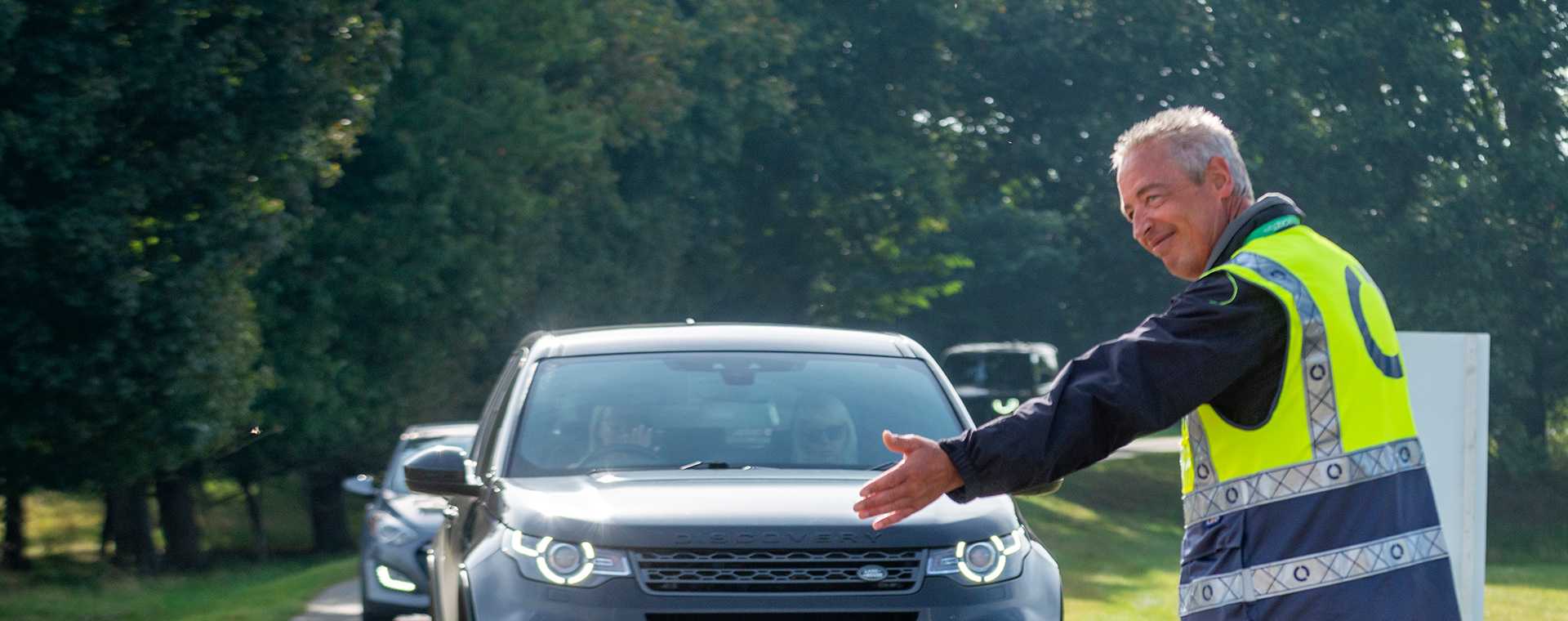The image depicts an older man with short whitish-gray, balding hair, wearing a long-sleeved dark blue jacket beneath a neon yellow and reflective gray safety vest. He is positioned on the right side of a small driveway or single-lane country road, his left arm extended outward, directing a row of slow-moving vehicles in the sunlight. He appears to be guiding a Land Rover, the first in line, possibly towards parking for an event, such as a wedding or concert. The background features lush green trees, through which sunlight filters, casting dappled light on the road and surrounding grass. The man has a slight smile or smirk on his face, adding a human touch to his role in managing the busy line of cars on what appears to be a very sunny day. The presence of right-hand drive vehicles suggests the scene is likely set in the UK.